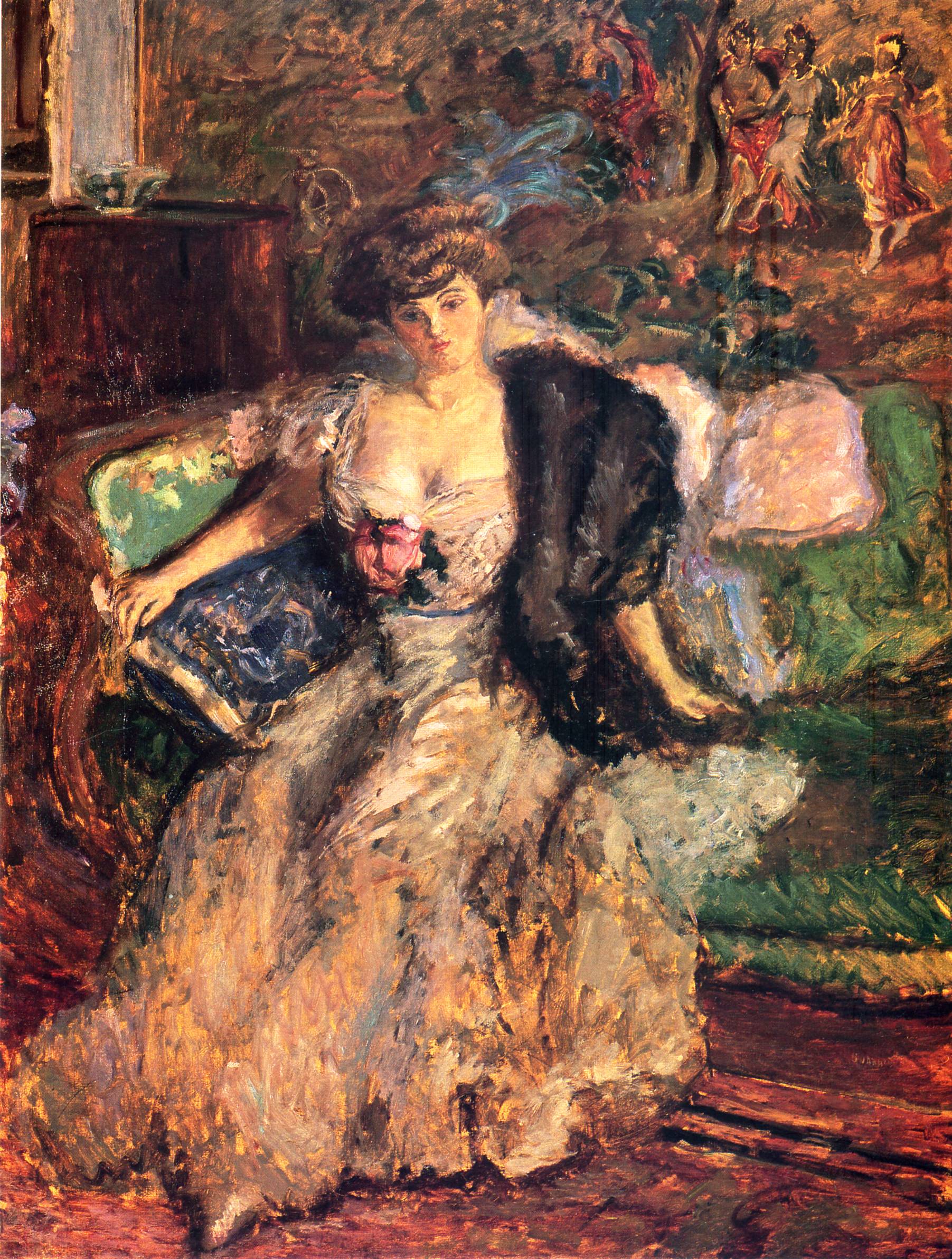This vertically aligned, rectangular image is a richly colored and highly detailed painting reminiscent of Victorian or Renaissance styles. At its focal point is an elegant woman with brown, curly hair styled in a coif. She gazes at the viewer with a serious expression, her lips closed and her upper chest exposed by a low-cut, white dress adorned with a pink rose on the bust. Draped over her left shoulder is a brown, possibly fur wrap, and her right arm is extended across the side of the green chaise sofa she is seated on. Under her right arm, a blue patterned throw pillow adds a pop of color. The ruffled bottom of her dress blends hues of light brown, gray, dark brown, and white, complementing the sofa. The background features a decorative wall with outlines of angelic figures and a dresser with a mirror on the back left. The predominant tones of dark browns and reds infuse the painting with a timeless, historical feel, further emphasized by intentional blemishes and slight blurriness, adding to its antique charm.